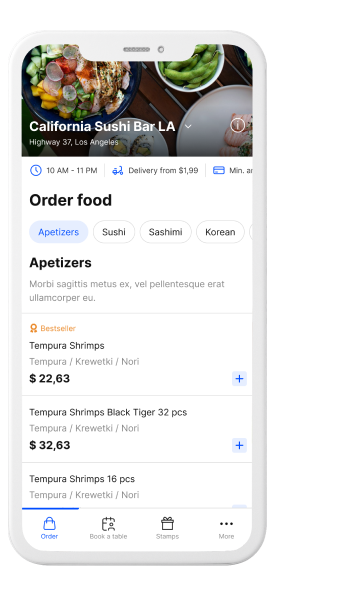**Descriptive Caption:**

The image showcases a detailed food menu advertisement for "Texas's California Sushi Bar LA," located near Highway 37 in Los Angeles. It prominently features a food bowl by Joe's, which contains a delectable assortment of veggies, protein, green beans, and sushi. Above the food bowl, there's a time indicator showing the operating hours from 10 a.m. to 11 p.m. Additionally, the advertisement mentions a vehicle resembling a scooter, used for deliveries starting from $1.99.

The menu highlights a variety of dishes including appetizers, sushi, sashimi, and Korean cuisines. Featured prominently is the bestseller – Tempura Shrimps, available in multiple options:
- Tempura Shrimp with Curry and Nori: 32 pieces for $32.63
- Tempura Shrimp with Curry and Nori: 16 pieces for $22.63

The menu also includes options to order food, book a table, and view more offerings, marked by various stamps and icons within the design.